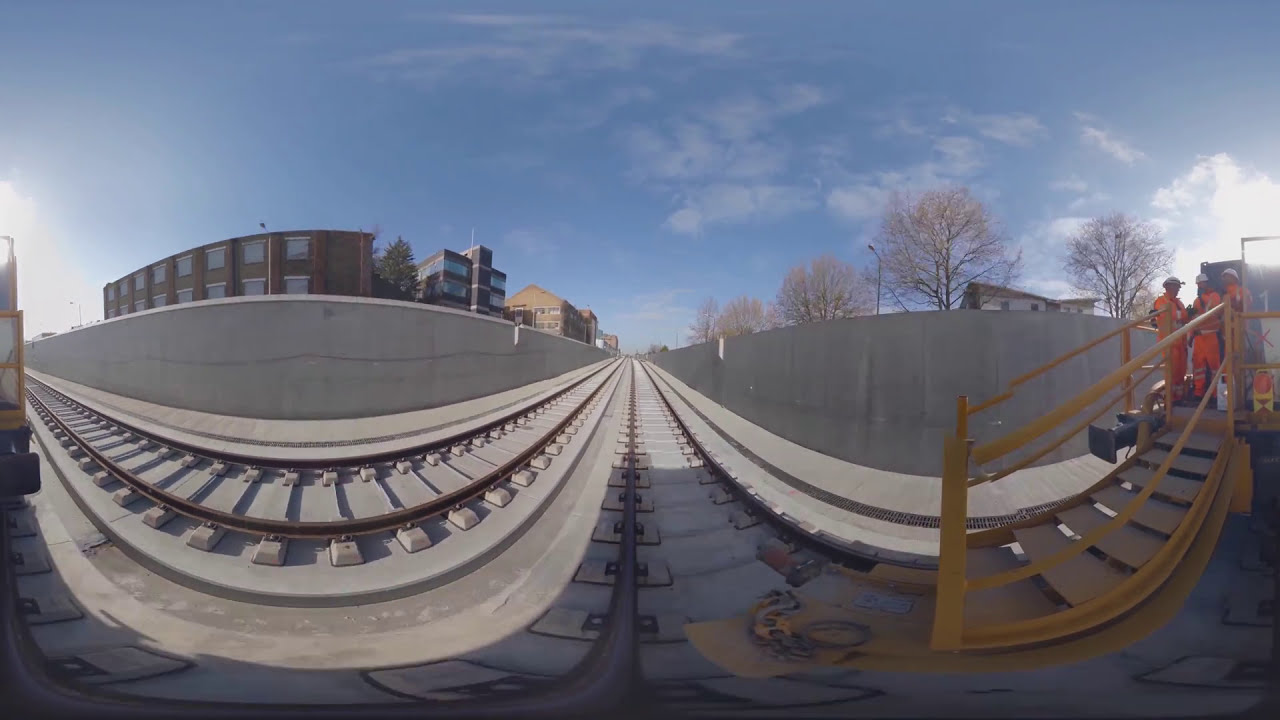The image portrays a distorted, high-angle view of a railway track, possibly captured with a 360-degree camera. The track runs through the bottom left quadrant, presenting a curvature due to lens distortion. To the right, the track appears to merge into a staircase with handrails. At the top of this staircase, three workers dressed in bright orange safety suits and white hard hats are visible. They seem to be conducting maintenance work. In the middle center of the image stands a concrete wall, extending partially out of frame. To the right of the wall, deciduous tree branches reach out against a backdrop of a partly cloudy sky. The image also shows a brown building with windows on the left side under a clear blue sky, and a noticeable sun flare in the left-bottom quadrant further accentuates the image's unique light effects, adding depth to the scene. The overall setting suggests an outdoor, industrial environment, mid-day.